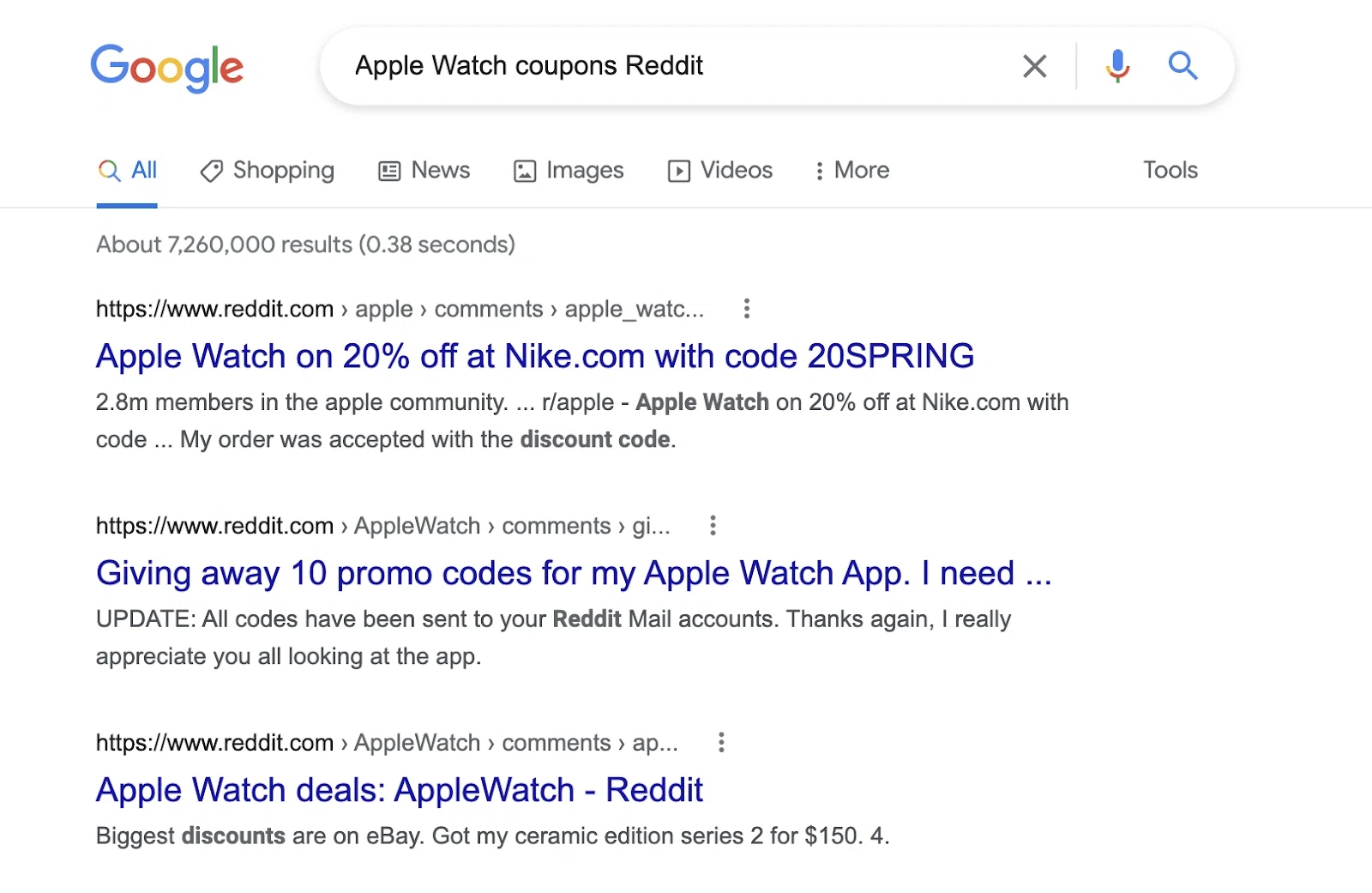Screenshot of a Google search page displaying results for "Apple Watch Coupons Reddit." The upper left corner showcases the familiar Google logo and brand name. Below, the search bar prominently displays the search query "Apple Watch Coupons Reddit." Beneath the search bar, a horizontal navigation menu features options such as "All," "Shopping," "News," "Images," "Videos," "More," and "Tools," all underlined in blue, with "All" currently selected.

The search results indicate approximately 7,260,000 results, retrieved in 0.38 seconds. The first result's URL is shown as https://www.reddit.com > apple > comments > apple_watch. This hyperlink, colored blue, reads "Apple Watch on 20% off at nike.com with code 20spring."

Below, in black text, it notes, "2.8 million members in the apple community... r/apple - Apple Watch on 20% off at nike.com with code... My order was accepted with the discount code." Another result immediately follows, offering 10 promo codes for an Apple Watch app, indicating their availability through Reddit mail. An update states, "All codes have been sent to your reddit mail accounts. Thanks again. I really appreciate you all looking at the app."

The next result, "Apple Watch deals apple watch - reddit," is highlighted in blue, mentioning, "Biggest discounts are on eBay. Got my ceramic edition series 2 for $150." This succinct text confirms the searcher's intent: finding Apple Watch coupons on Reddit.